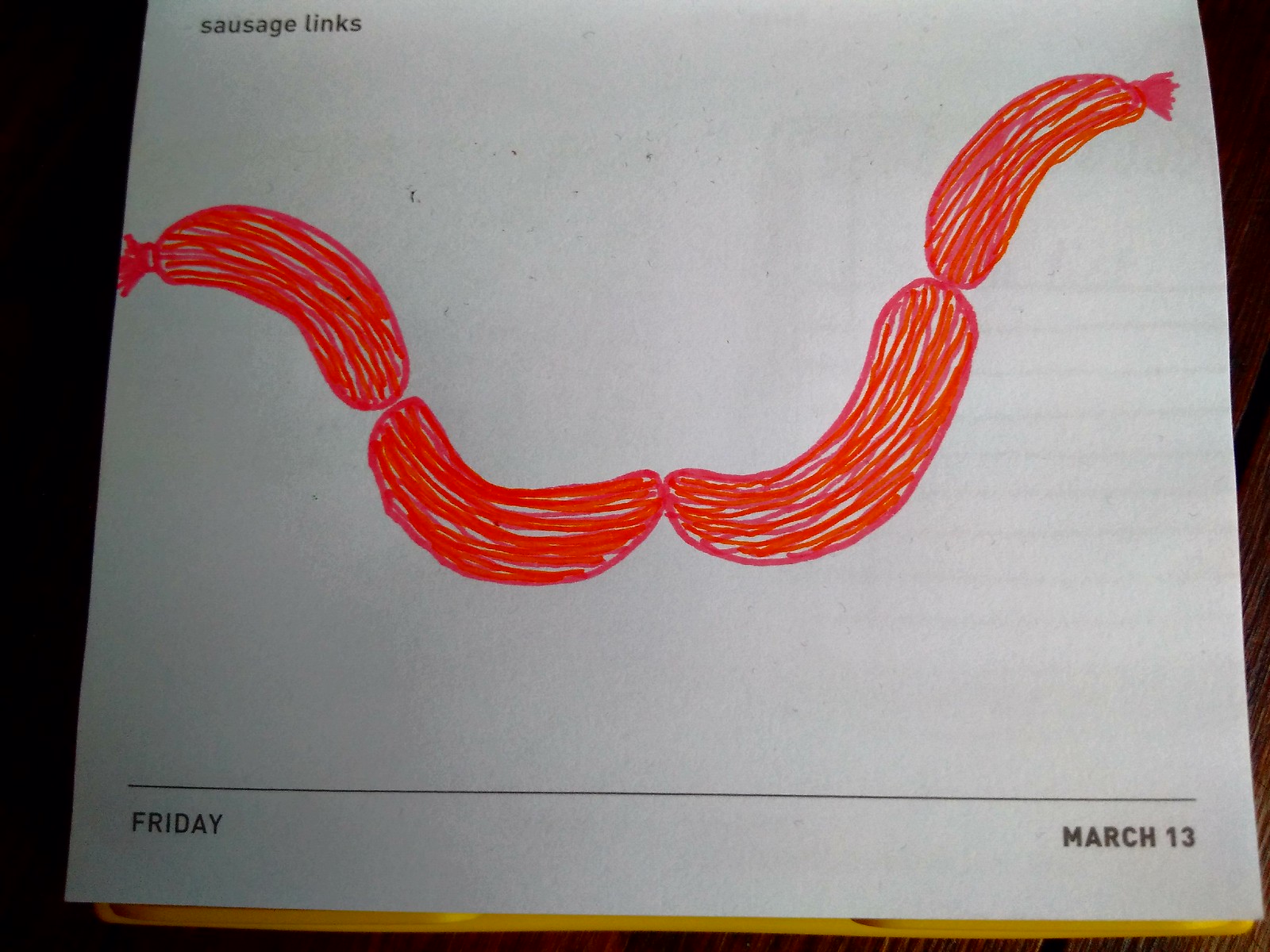The image portrays a page from what appears to be a daily tear-off calendar, predominantly white in color. Centered on the page is a hand-drawn illustration of four red sausage links forming a loose U-shape with visible white gaps where the red coloring is incomplete. The sausages are lightly scribbled in a mix of red and orange, resembling a playful doodle. Black text in the upper left corner labels the drawing as "Sausage Links." At the bottom, aligned with the thin black divider line above, the page is marked with the day "Friday" on the lower left and the date "March 13th" on the lower right. The white page appears to be set against a black background, with a hint of something yellow possibly serving as a base or frame beneath it.